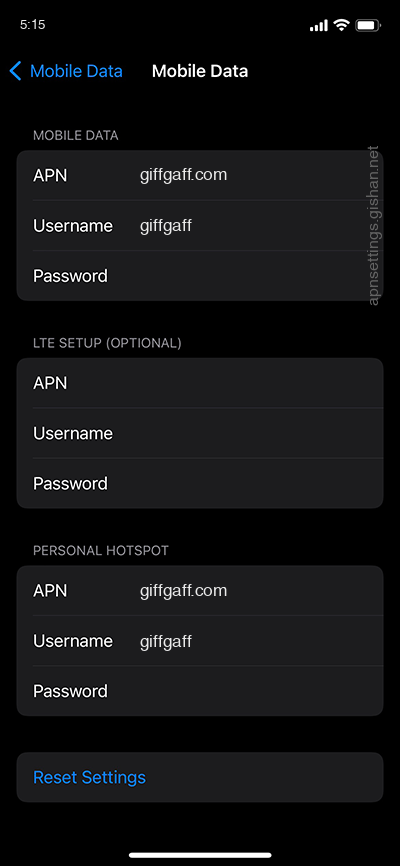This is a highly detailed screenshot of a smartphone's settings interface, captured against an all-black background. At the top left, the screen displays the current time as 2:40. On the top right, there are two internet connectivity icons, alongside a mostly full battery indicator. Below this, the text "Mobile data" appears twice: on the left in blue with a blue caret pointing left, and on the right in white.

The interface is divided into four main categories:

1. **Mobile Data:**
    - **APN:** GIFFGFF.com
    - **Username:** GIFFGFF
    - **Password:** (not displayed)
    - To the right of the username and password fields, there is a line of text indicating "APN settings" from GISHAN.net.

2. **LTE Setup (Optional):**
    - **APN:** (blank)
    - **Username:** (blank)
    - **Password:** (blank)

3. **Personal Hotspot:**
    - **APN:** GIFFGFF.com
    - **Username:** GIFFGFF
    - **Password:** (blank)

4. At the very bottom, there is a blue button labeled "Reset Settings."

This well-organized layout allows users to easily navigate and configure their mobile data and personal hotspot settings.